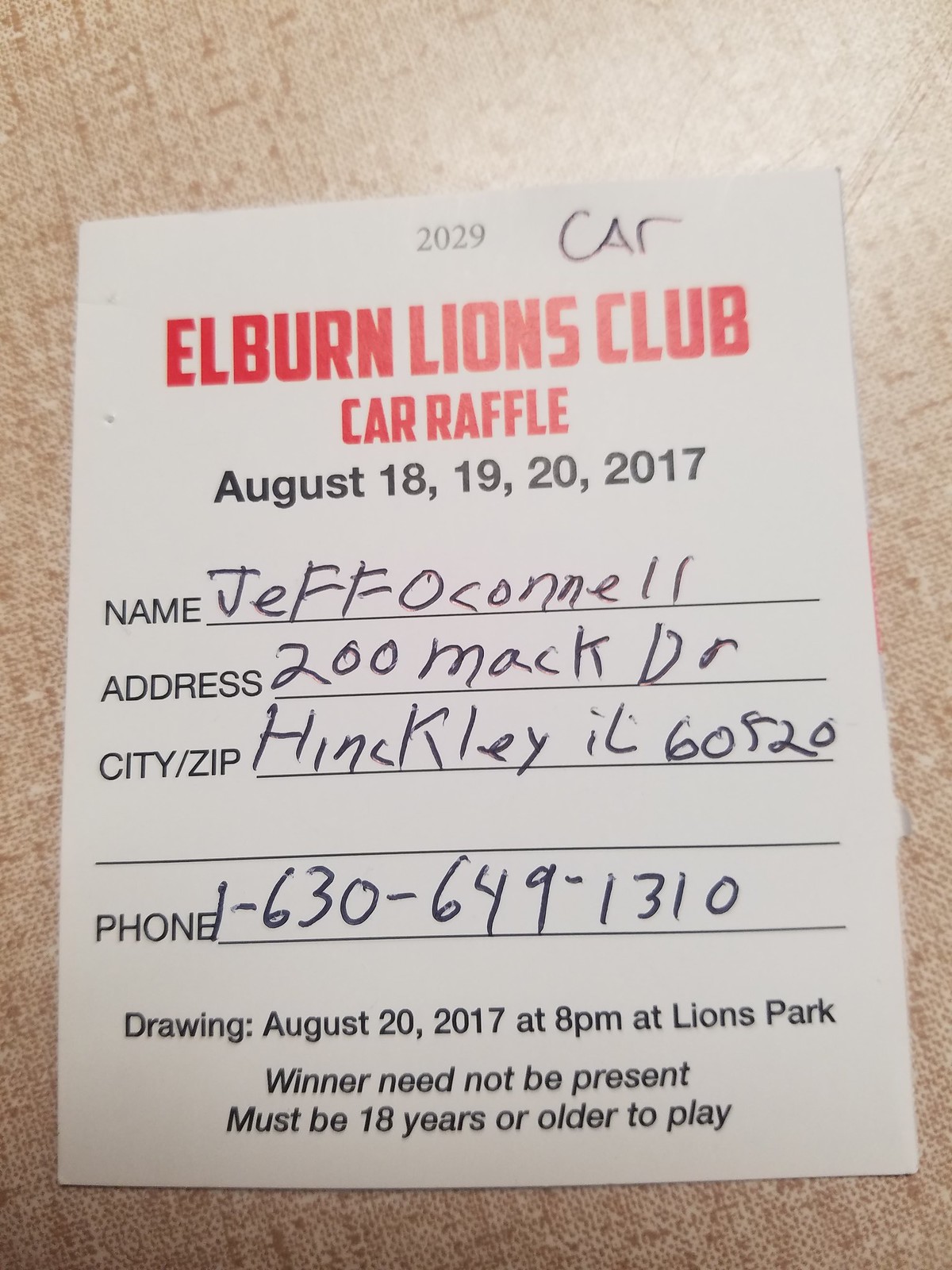The photograph features a small white raffle ticket placed on a beige cloth, possibly a couch. The ticket, titled "Elburn Lions Club Car Raffle," has various text details in black and red fonts. At the very top, the number "2029" is printed in black, and "CAR" is handwritten next to it in black ink. Below, in red font, "Elburn Lions Club Car Raffle" is prominently displayed, followed by "August 18, 1920, 2017" in black font, which seems to be a typographical error. The ticket includes personal information such as the name "Jeff O'Connell," address "200 Mack Drive," city/zip "Hinckley, IL 60520," and phone number "1-630-649-1310," all handwritten. The lower section details the drawing information: "Drawing: August 20, 2017 at 8 p.m. at Lions Park. Winner need not be present. Must be 18 years or older to play." The colors present in the ticket's text are black and red, set against the white paper, with the beige cloth serving as the backdrop.